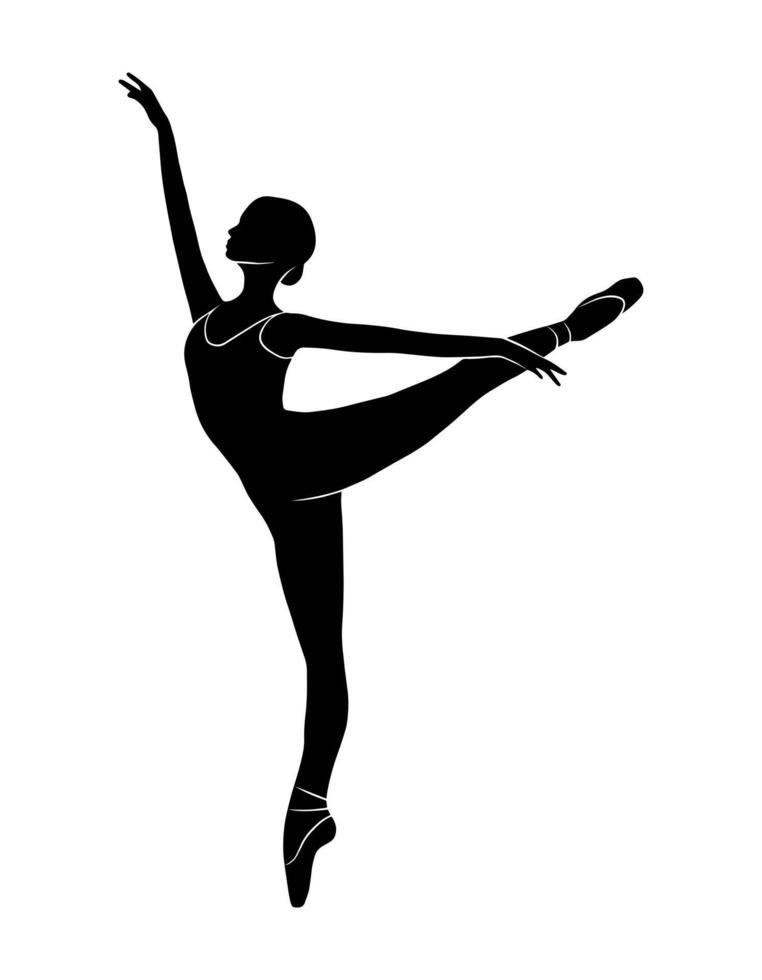This black and white image, resembling a detailed sketch, features a silhouette of a ballerina set against a solid white background. The ballerina is entirely black, with white edging used to accentuate various parts of her form, lending clarity to her graceful pose. She stands en pointe on her right foot, with her toes delicately touching the ground and her heel raised, highlighting her right ballet shoe with a white outline. Her left leg is extended behind her at an angle slightly higher than 90 degrees, also en pointe with white marks depicting the ankle tie and the tip of the shoe. 

Her right arm reaches elegantly upwards while her left arm stretches out behind her at a 90-degree angle. The ballerina’s head is tilted slightly back, with a small bun visible. She is clad in a skin-tight tank top leotard, its shape and neckline subtly defined by white lines around the shoulders and neck, as well as creases near her ankles that suggest the leotard extends down her legs. The overall simplicity of the color scheme, combined with the precision of the white details, creates a striking and sophisticated silhouette, perfect for use in various visual applications like t-shirts or advertisements.